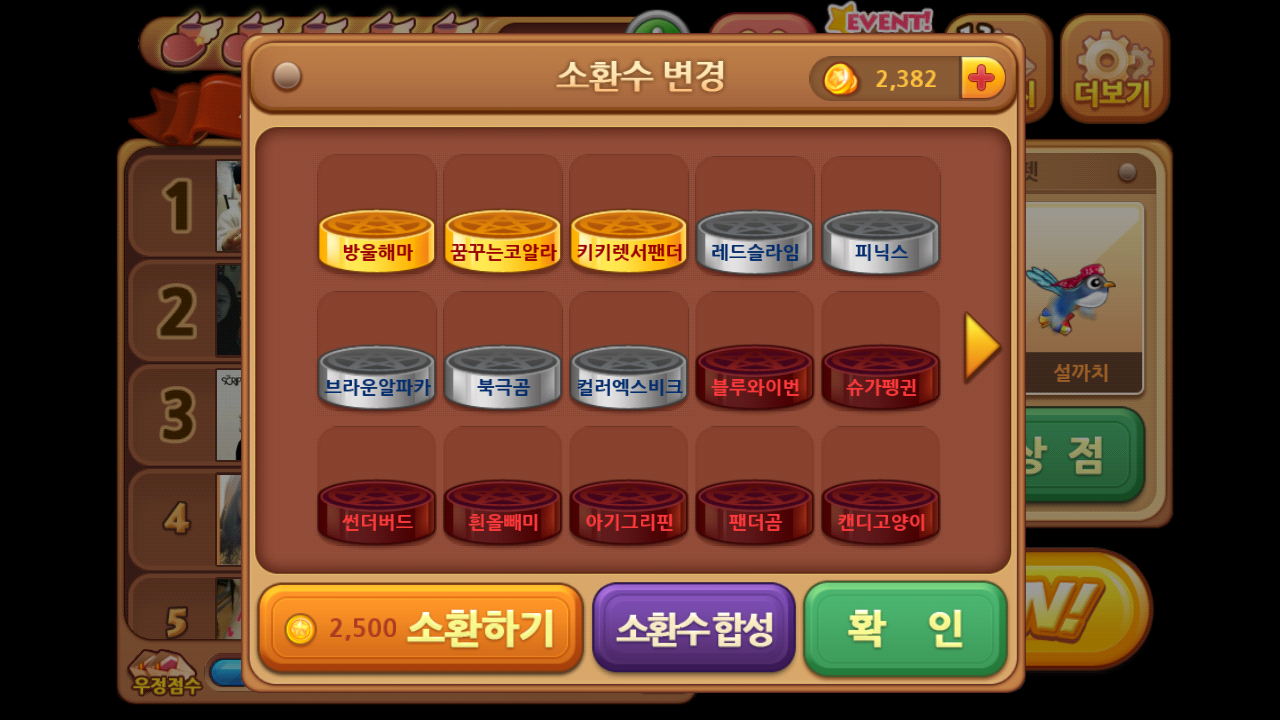This image depicts a screen from an Asian digital slot machine game, potentially Japanese. The foreground features a grid of coins arranged in three rows. The top row contains three golden coins followed by two silver coins, all marked with Chinese characters. The middle row shows three silver coins and two dark red coins, each also featuring Chinese characters. The bottom row consists of five dark red coins with matching characters. Below this grid, there are three buttons: a golden button with Chinese characters and the number 2,500, a purple button with white Chinese characters, and a sea green button with white Chinese characters.

In the background, there's another screen partly obscured by the foreground elements. This background screen includes columns or rows labeled one through five, and a small bird wearing a hat is visible on the right-hand side. 

Additional details include a box in the top right showing the player’s total of 2,382 tokens. The numerical and textual interface elements are solely in Chinese characters, and it appears that the player does not have enough tokens (2,382 versus 2,500) to make a purchase or win the required amount.